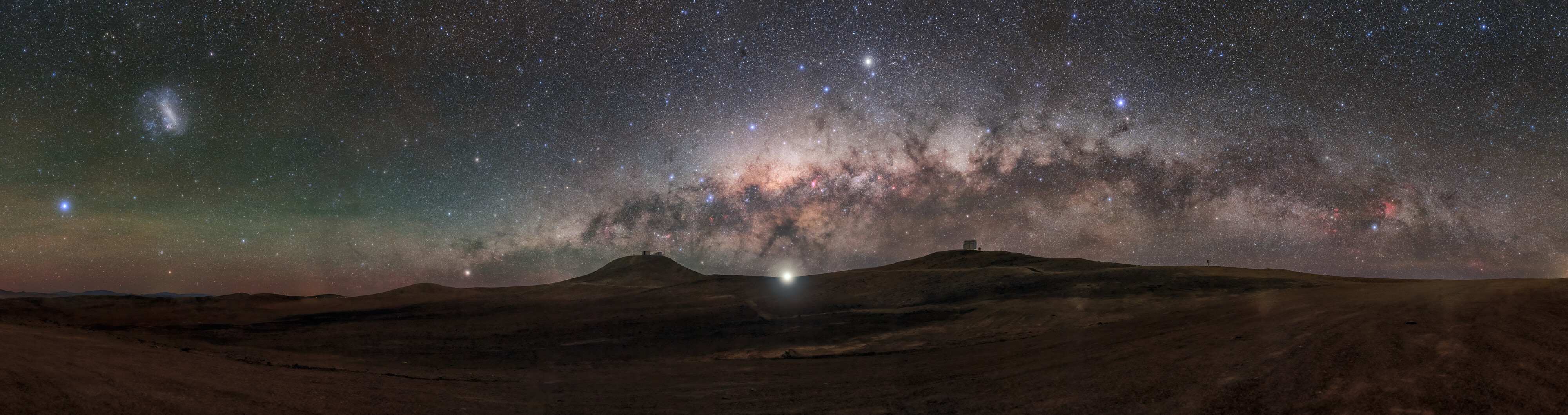This wide, horizontally expansive landscape image, captured during nighttime, depicts an otherworldly scene that merges elements of a desert and a mystical sky. The lower third of the image is dominated by darkened hills or dunes, resembling a desert landscape with a texture and color suggesting dirt. Above these hills, the sky defies earthly expectations, blending cosmic and aurora borealis elements in a mesmerizing display. The right side of the sky features a chaotic spread of starry, cosmic light, reminiscent of a view through the Hubble telescope, while the left side reveals an aurora-like display with hints of pinks, greens, and blues. Strands of glistening, smoke-like clouds add to the surreal atmosphere, along with intermittent flecks of light that appear like stars. The photograph conveys a sci-fi, outer space aesthetic, presenting a contrast between the stark, isolated landscape below and the enchanting, almost magical celestial display above.